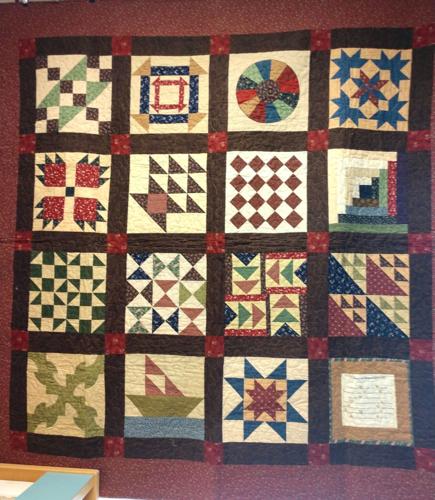The image depicts a richly detailed, handmade quilt or wall hanging, characterized by its grid pattern of intersecting squares, 4 by 4 in total. The background is predominantly a deep burgundy color, reminiscent of dark wood. Each square in the grid is bordered by brown frames, with the intersections featuring smaller red squares adorned with yellow prints, creating a layered, nailed-on effect.

Inside each framed square, the backgrounds vary in hues but are predominantly yellow, serving as canvases for various geometric shapes and intricate designs. Among the numerous patterns, you can spot a pie chart, a boat made out of triangles, checkered spots, leaf or feather-like motifs, and diamond configurations. One square near the bottom right corner even contains handwritten text, adding an element of personal touch to the overall design. The quilt showcases a myriad of colors and patterns, combining the meticulous craftsmanship of sewing with artistic flair, resulting in a vibrant, visually intricate piece.